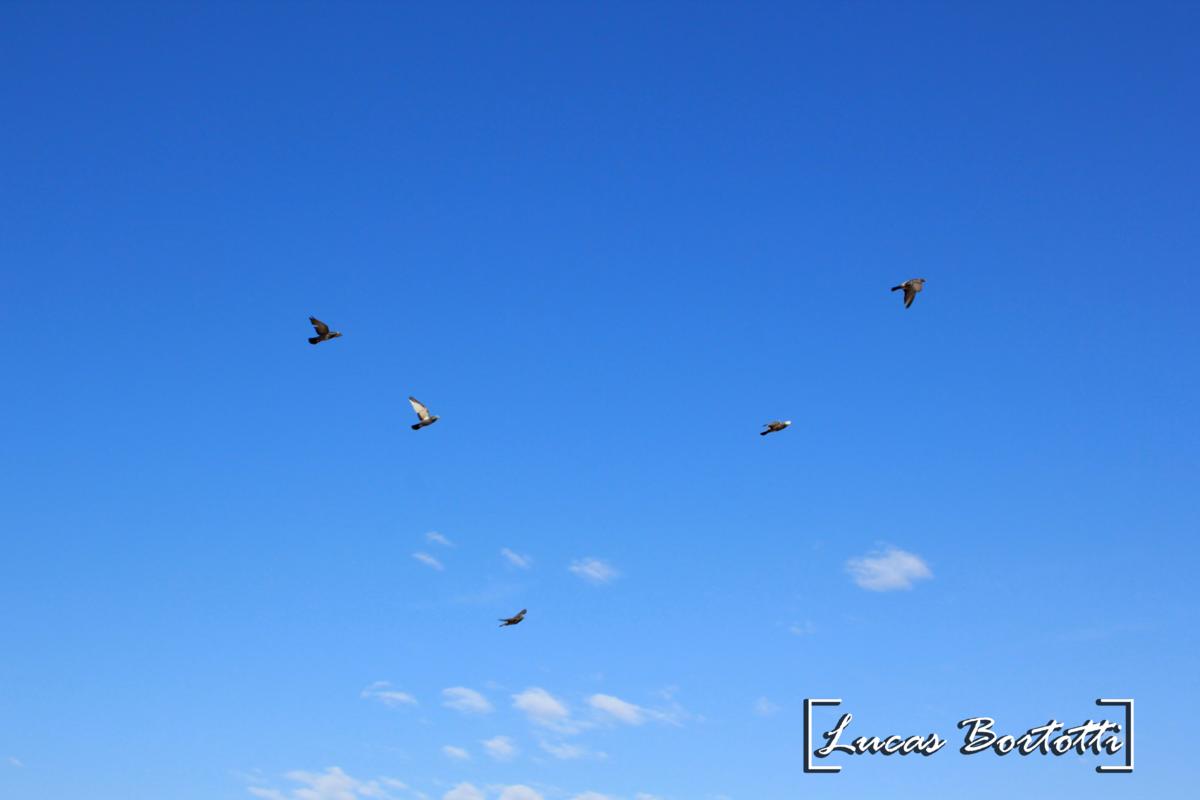The image is a horizontally oriented, realistic color photograph taken outside during the day, featuring a brilliantly blue sky that deepens in tone from top to bottom. Along the bottom of the sky, small, fluffy white cirrus clouds are visible. Five dark brown or black birds, possibly eagles or another type of bird of prey, fly in a V-formation towards the right, with one bird exhibiting a white underwing. Notably, one bird appears to have a white head. In the bottom right corner of the image, there is a signature and logo in square white brackets with a black outline, written in white script with a black outline, reading "Lucas Bortotti."